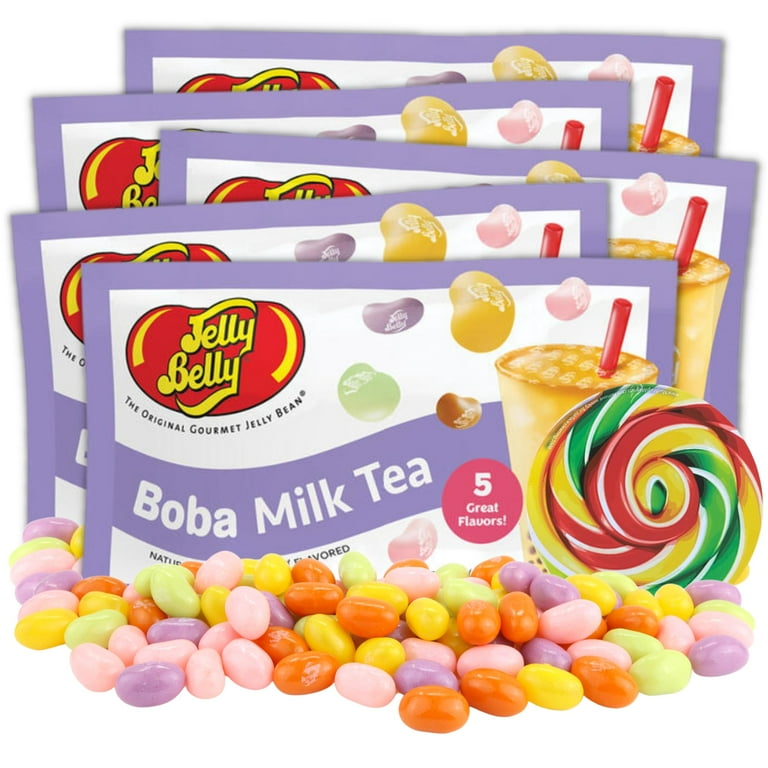This image features multiple packages of Jelly Belly, the original gourmet jelly bean, in a boba milk tea flavor. The packaging is predominantly white with a purple border and a purple banner across the middle, which features "Boba Milk Tea" written in white text. In the upper left corner of each package, there is a red jelly bean-shaped oval with "Jelly Belly" written in yellow text and "The Original Gourmet Jelly Bean" in smaller black font beneath it. The bottom right of the package showcases a pink circle with white text announcing "Five Great Flavors," accompanied by an illustration of a milk tea glass with a red straw.

Scattered around the bottom of the packages are various colored jelly beans, including pink, purple, orange, yellow, and light green, showcasing the diversity of flavors included. Despite the boba milk tea theme, the jelly beans come in an array of colors not typically associated with the drink. The packages also display representations of the jelly beans, which highlight the unique and colorful assortment.